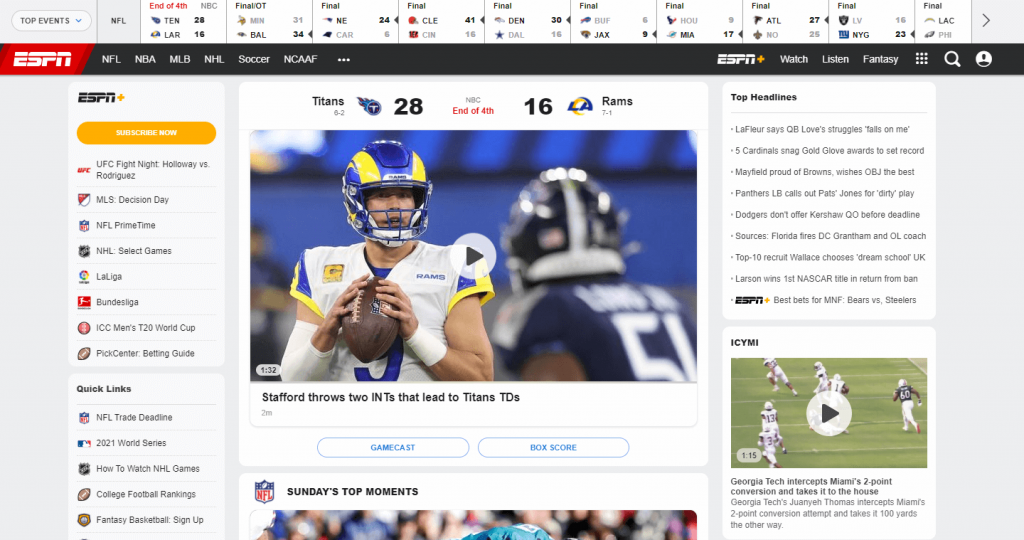This image is a detailed screenshot of ESPN's website showcasing sports news and updates from a specific period. The navigation bar at the top of the webpage provides quick access to various sports categories, including NFL, NBA, MLB, NHL, Soccer, NCAA Football, and more. 

Visible on the bar are the latest scores and game results: Tennessee nailed a 28-16 victory over the Rams, Baltimore edged out the Dolphins with a close 33-30, Cleveland dominated the Bengals 41-16, and Jacksonville surprisingly defeated Buffalo 9-6 in what must have been a frigid game. Atlanta narrowly triumphed over New Orleans with a 27-25 score. The Las Vegas Raiders initially seemed to have won against the Giants, but the correct score reveals a 23-16 victory for the Giants instead. The Chargers managed to outperform the Eagles, though the exact score is unclear.

On the left side of the website, multiple sections such as NFL Primetime, NHL games, and UFC Fight Night provide additional coverage and updates. The main content section is dedicated to the Titans-Rams game, which ended with a score of 28-16 in favor of the Titans. A noteworthy highlight is Matthew Stafford's two critical interceptions that led to Titans' touchdowns; however, despite this, the Rams went on to win the Super Bowl that year.

Below the main content, the page features sections like "Sunday's Top Moments," highlighting key plays and game recaps from various sports events. The page layout is designed to offer quick access to the latest sporting news, highlights, and scores.

At the very top of the page, headlines include Kyle Larson's remarkable comeback to win his first NASCAR title after a suspension for using a racial slur on a Twitch stream. Other headlines note that the Dodgers did not extend an offer to pitcher Clayton Kershaw before the deadline and a Panthers linebacker called out the Patriots for dirty play, inviting no surprise.

This comprehensive setup encapsulates the dynamic and extensive sports coverage ESPN provides.